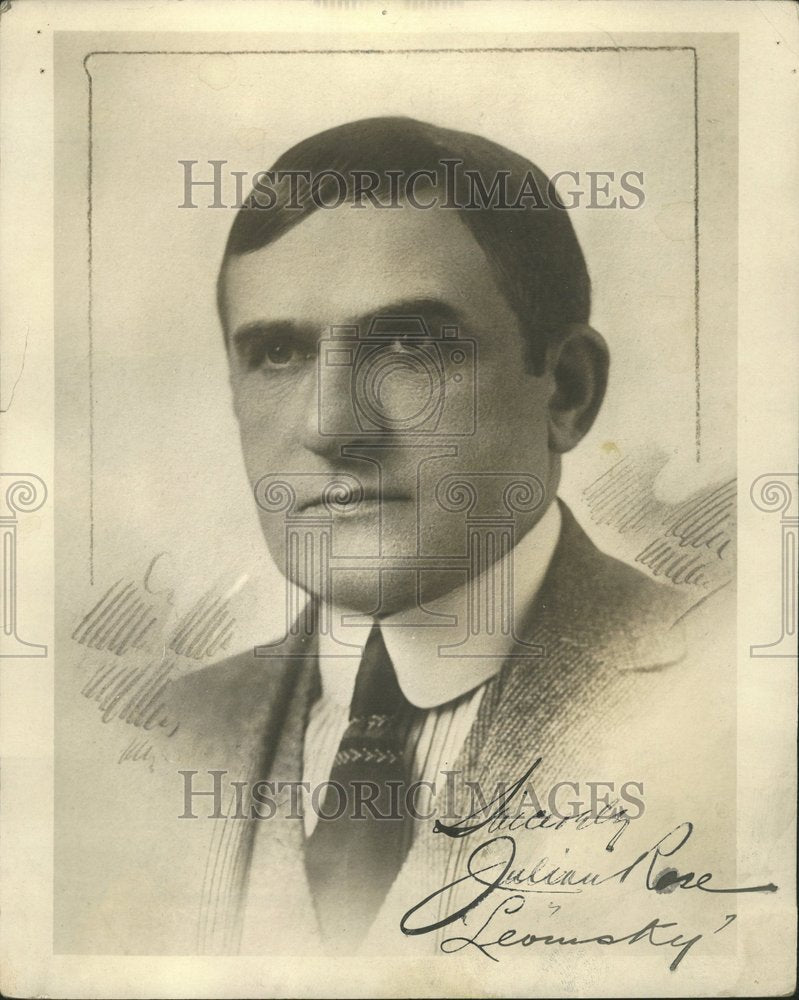This is a vintage black-and-white photograph of a solemn-looking man, likely in his mid-30s, with slick, short brown hair combed over to the right. The paper shows its age with a yellowed appearance and watermarks at the top and bottom reading "Historic Images." The watermark design includes three pedestals of varying heights with a camera atop the tallest middle pedestal. The man’s expression is stoic and he gazes slightly to the left, not smiling. He wears a white collared shirt with vertical stripes, a darker tie featuring an arrow pattern, and a vest underneath a tweed-style jacket. At the bottom right corner, the photograph is signed in cursive, seemingly reading "Sincerely, Julian Rose LaVestie," although there is some variation in interpretation. The drawing-like quality of the image creates a cream and gray modeled background that fades toward the bottom.